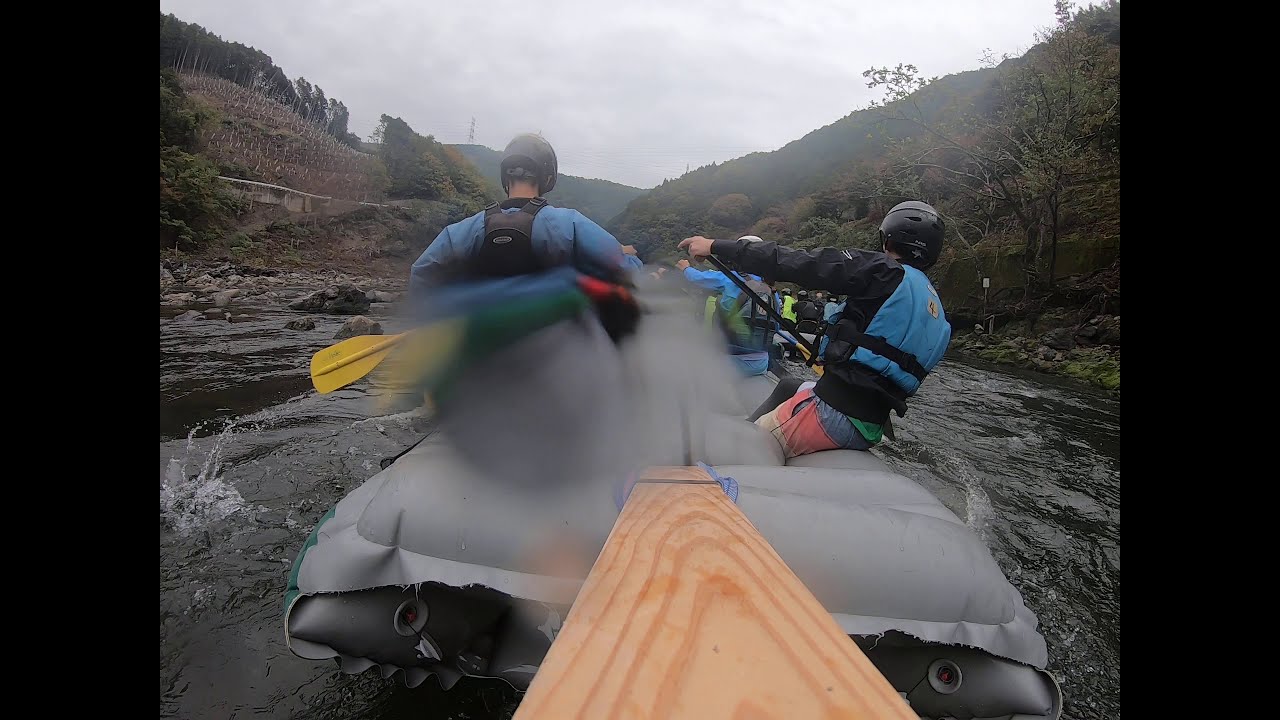A gray inflatable raft is navigating a river, with two visible rafters on its outer sides. The raft features a darker gray center with lighter gray sections and black objects towards the underside. A board is affixed to the back of the raft with a blue string. The individual on the left wears a blue jacket, black helmet, black safety vest, and holds a paddle with a yellow oar. Meanwhile, the person on the right, leaning towards the right side, is dressed in a black long-sleeved shirt, black helmet, blue safety vest, and colorful shorts with shades of red, orange, yellow, and blue. He grips the edge of a black paddle. Further ahead, a few more people can be seen. The landscape shows the slopes of tree-cleared mountainsides on the left, with the right side featuring large, rounded rocks protruding from the river. The dark water below has visible ripples. In the far distance, an antenna tower caps the mountain slope, all beneath a heavily clouded sky with mixtures of white and gray. This scene captures the essence of a challenging whitewater rafting adventure on a cloudy day amidst rugged, tree-sparse mountains.